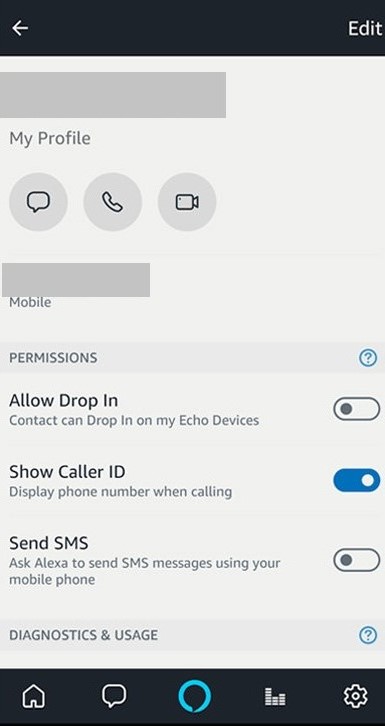The image showcases a mobile interface with a tall, screen layout. At the top of the screen, there's a dark area with a white arrow pointing to the left and the word "Edit" in white text on the right. Below this section, there is a gray page with various elements.

In the upper left corner of the gray page, a darker gray box covers part of the content. Directly below this, the text "My Profile" is displayed in gray. Underneath "My Profile," there are three circular icons aligned horizontally: a speech bubble icon on the left, a phone icon in the middle, and a camera icon on the right.

Further down, there's another gray box with the word "Mobile" beneath it. Following this is a titled section "Permissions" which includes a blue question mark enclosed in a circle. Under this heading, several settings are listed:

1. **Allow Drop In:** A setting for contacts to drop in on Echo devices, currently switched off.
2. **Show Caller ID:** A setting to display the phone number when calling, which is turned on, indicated by a blue button.
3. **Send SMS:** A setting that allows Alexa to send SMS messages using the mobile phone, which is turned off.

At the bottom, there's a section labeled "Diagnostics and Usage." Finally, the bottom-most part of the interface features a black area containing various icons.